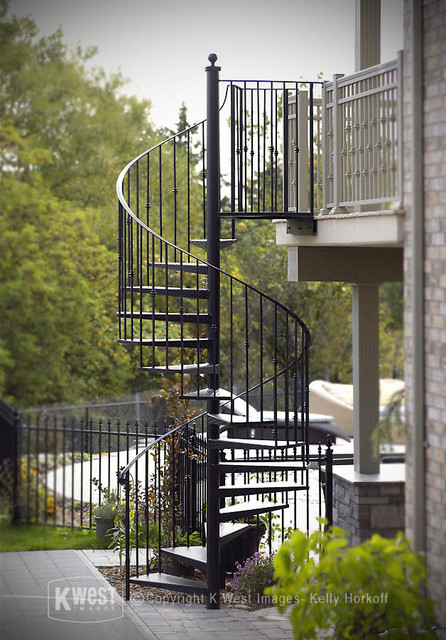This is an exterior photo featuring the side of a house with a distinct black iron spiraled staircase that wraps gracefully around a single metal pole, leading up to a second-floor balcony. The house itself has a sophisticated facade made of cream and gray bricks. The balcony, adorned with white metal railings that showcase a delicate diamond pattern, adds a touch of elegance. Below the balcony, a thin T-column and a broader brick column suggest a well-thought-out architectural design. In the foreground, a small green plant is visible, complementing the cement area that stabilizes the winding staircase. Further behind the house, a black metal fence with individual spikes encloses a section that possibly contains a man-made rockery or a similar structure, painted white. The background reveals lush green trees, indicating a non-urban, tranquil setting. A piece of garden furniture is also visible amidst the greenery, adding to the serene outdoor atmosphere. The image bears the credit "K. West images," attributed to Kelly Horkoff.